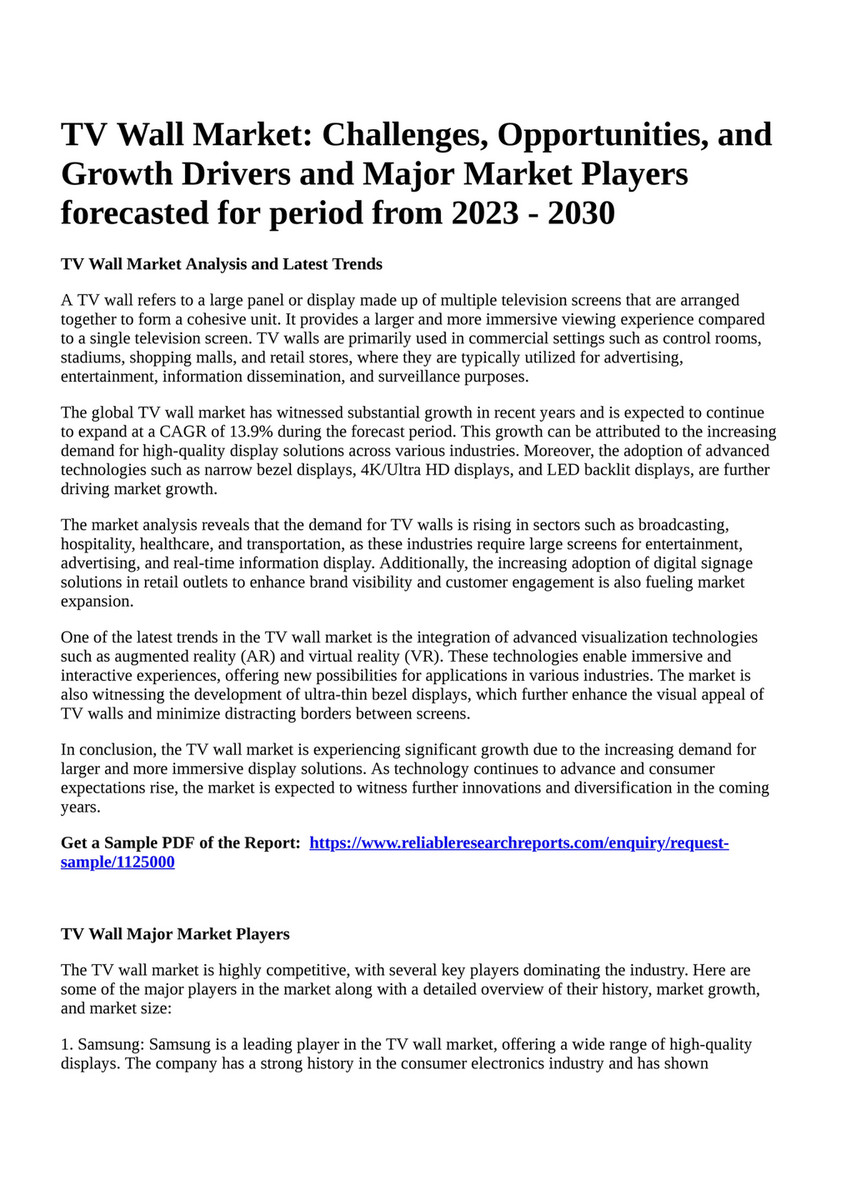The image depicts a section of a detailed report against a white background, headlined with bold black text that reads, "TV Wall Market: Challenges, Opportunities, and Growth Drivers and Major Market Players, Forecasted for the Period from 2023 to 2030." Below this, in a smaller bold font, it says, "TV Wall Market Analysis and Latest Trends." The body of the document contains five left-aligned paragraphs of informative text. The first paragraph begins by defining a TV wall as a large display made up of multiple television screens arranged cohesively. Further down, there is a bold line inviting readers to "Get a sample PDF of the report," followed by a clickable blue link. Following this, another bold section titled "TV Wall Major Market Players" leads into two additional paragraphs of content.